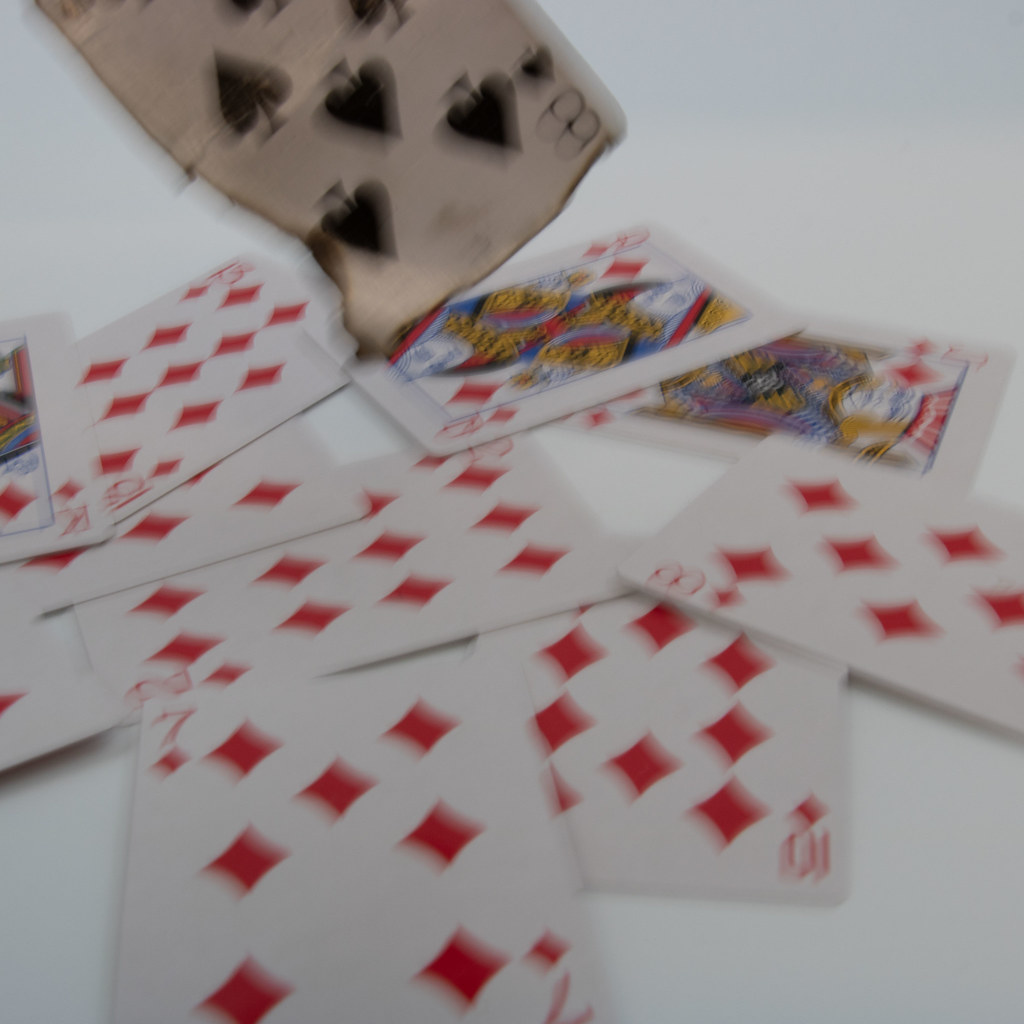The image features a collection of playing cards scattered across a white surface, which might be a table or desk. The photograph is notably blurry, making it challenging to distinctly identify all the cards. At the top of the image, there is an 8 of Spades card that stands out due to its burnt, darkened appearance with singed edges, adding a focal point of intrigue. Below this burnt card, towards the center and background of the image, lie additional cards, primarily from the Diamonds suit. Notably among them are a Queen of Diamonds and a King of Diamonds, albeit their details are obscured by the blur. A 7 of Diamonds is also discernible. The cards are haphazardly arranged, some overlapping each other, but the burnt 8 of Spades remains the most compelling and visually distinctive element in the composition.